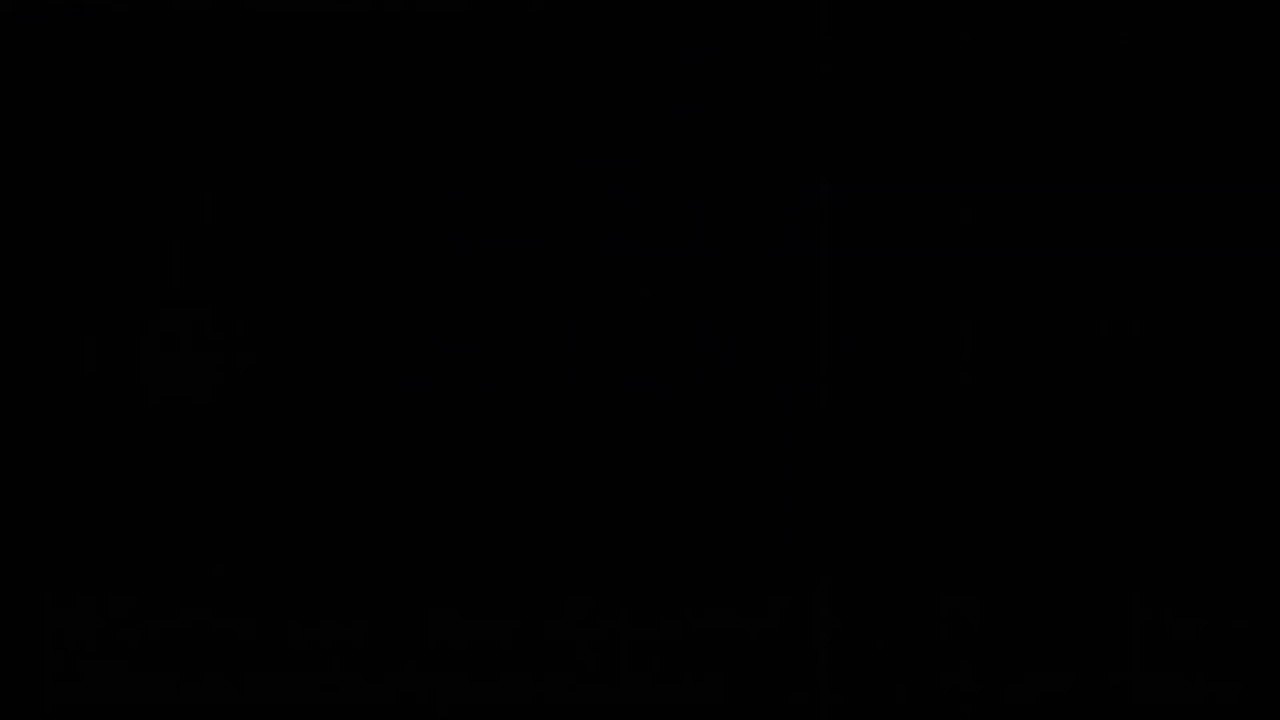The image depicts a solid black rectangle that is twice as wide as it is tall, approximately 8 inches in width and 6 inches in height. The rectangle contains no visible elements, colors, or objects, and it gives an impression of complete void or emptiness, akin to the vastness of space or perhaps even a black hole. There are no signs of ads, videos, or any interactive content within the frame. It's just an unbroken expanse of darkness that prompts contemplation on various black things, from black licorice to black cats, and symbolizes pure nothingness.